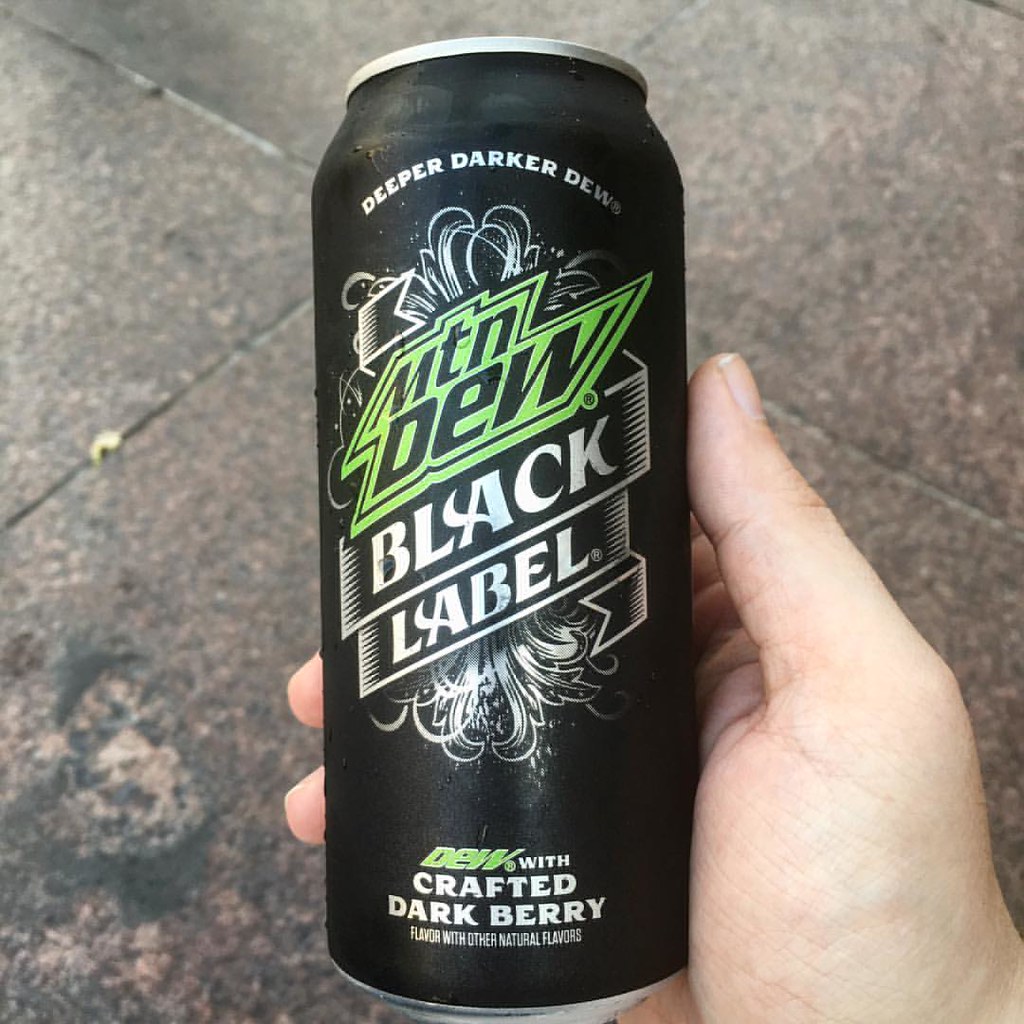This photograph features a Caucasian male's right hand, visible from the thumb's bulge upwards, holding a black can of Mountain Dew Black Label against a concrete floor. The can has a silver top and is adorned with an intricate, almost Victorian calligraphy style design, resembling fireworks. In white at the top, the can reads "Deeper Darker Dew". A green lightning bolt runs across the upper section, with "Mountain Dew" inscribed in black within the bolt. Below this, "Black Label" is printed in white against a black background with pointy decorations and swirling lines. At the very bottom, "Dew" is written in green, followed by "Crafted with Dark Berry" in smaller white text. The floor in the background appears to be a concrete surface, possibly made of stone tiles or sections, showing visible lines and wear, akin to a gymnasium or a sidewalk.